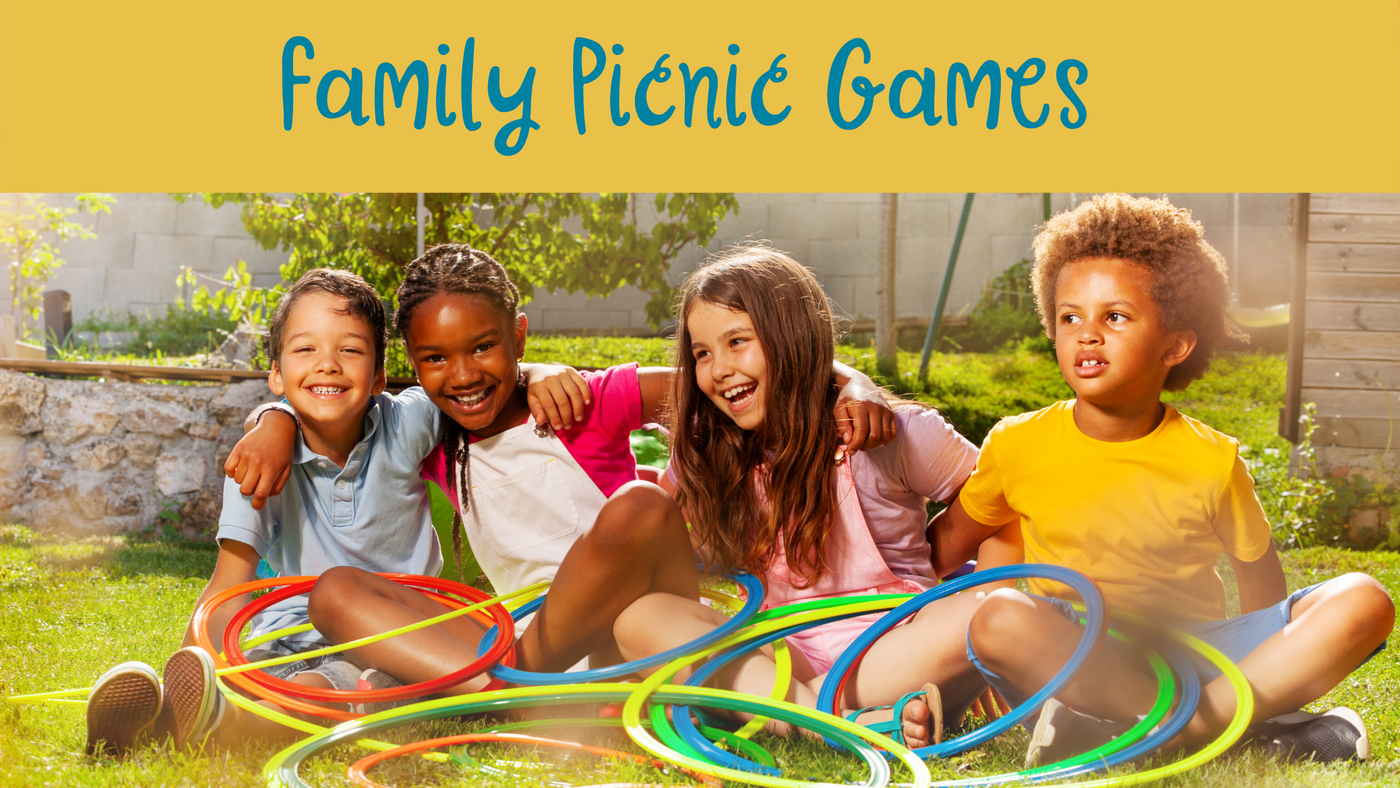The image is an advertisement for family picnic games. At the top, there is a goldish-colored banner with "Family Picnic Games" prominently displayed in blue print. Below the banner, the scene is set outdoors, likely in a backyard or school ground, featuring a backdrop of a white cylindrical stone wall and a green tree with low branches.

In the foreground, four children, two boys and two girls of different ethnicities, sit cross-legged on a grassy area. They are wearing colorful clothing and shorts. The children have several colorful hula hoops or rings in their laps and have their arms around each other, giving the impression of camaraderie and happiness. Two of the children are looking directly at the camera, while the other two gaze to the left of the image. The overall atmosphere is cheerful and engaging, highlighting the fun of family picnic games.